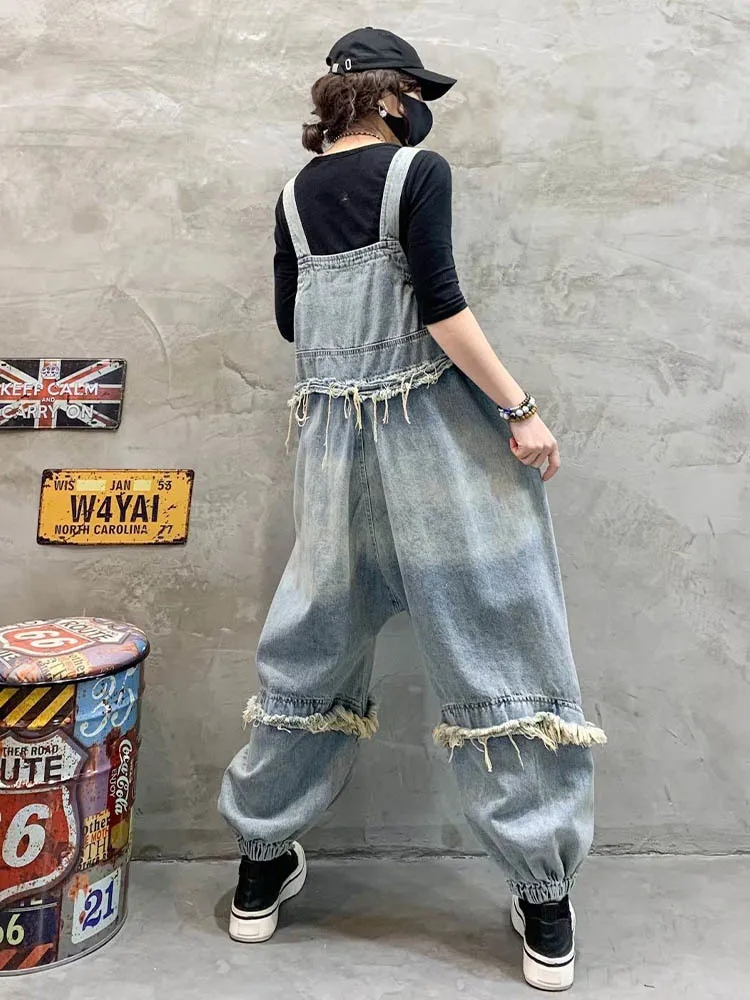The photograph depicts a person, presumably a woman, standing in front of a grey, cement-like wall with a distinctive, textured pattern. She is central in the image, standing with her body facing slightly towards her right. The woman is wearing a black baseball cap, a black face mask, and has short brown hair tied into a small ponytail at the nape of her neck. Her attire consists of a black top with elbow-length sleeves and denim dungarees that feature frayed edges at the waist and knees, giving them a slightly frilled effect. The dungarees are gathered at the ankles by elastics, and she is sporting black and white sneakers with thick soles. On her right wrist, she wears a beaded bracelet.

To her left, affixed to the wall, are several metal license plates and other memorabilia. One license plate features the British Union Jack with the phrase "Keep Calm" on it, and another is a yellow plate with the inscription "WAW4YAI." Below these is a painted oil drum adorned with various signages, including the numbers "66" and "35," the iconic Route 66 symbol, and a Coca-Cola logo, complemented by yellow and black chevrons. The background's array of Americana elements contrasts with the simplicity of her outfit, creating a visually striking composition.